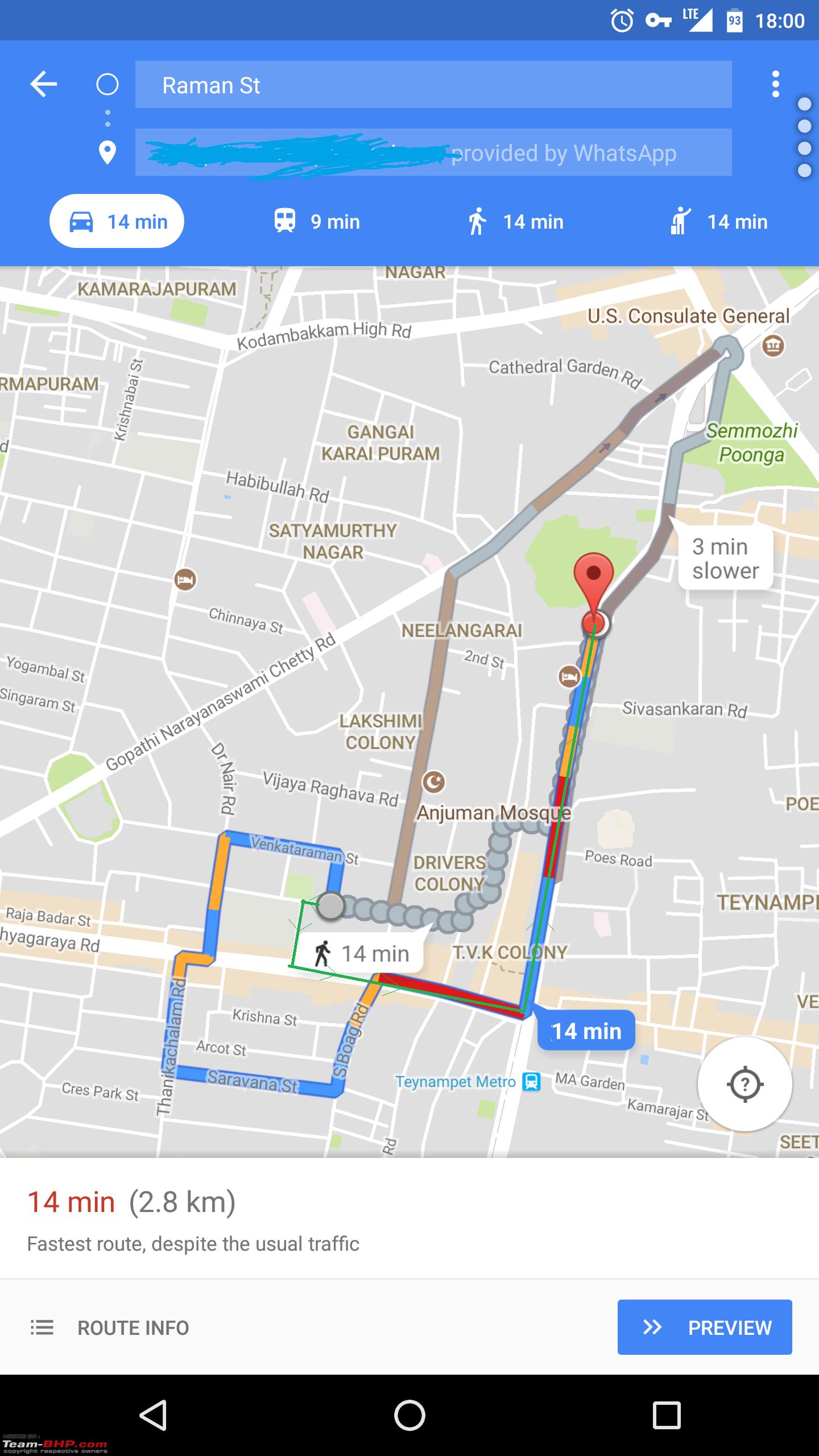The image is a detailed screenshot of a Google Maps navigation interface displayed on a mobile device. At the very top of the screen, there is a dark blue status bar featuring several white icons. These include an alarm icon, a key icon, an LTE connection symbol, a battery indicator showing 93% charge, and the time displayed as 18:00 (6:00 PM). Directly below this, the background transitions to a lighter but still prominent blue, which houses the Google Maps user interface.

Starting from the top of the Google Maps UI, there are two light blue rectangles. The upper rectangle is labeled "Ramen Street," indicating the starting location. The lower rectangle has partially obscured information where dark teal digital markings cover part of the text. The visible portion reads "provided by WhatsApp." To the left of these rectangles are three icons: a circle, a location pin, and a left-pointing arrow.

Below this, an oval button highlighted in white shows "14 minutes," suggesting the current selected route's duration. To the right are alternative route options: a train (9 minutes), walking (14 minutes), and presumably a taxi, illustrated by an icon of a man with a suitcase (also 14 minutes).

Further down, there is the actual map image, followed by additional UI details on a white background. It indicates the selected route's duration in red ("14 minutes"), distance ("2.8 kilometers"), and a note claiming "fastest route, despite the usual traffic." Underneath, there is a navigation bar with a brief route info menu icon on the left and a blue "Preview" button with two rightward arrows on the right.

At the very bottom, the phone's native navigation controls are displayed: a back symbol, a circle, and a square. In the bottom left corner of the screen, there is a small, stamped text that reads "team BHP com" in white and red letters, though the rest of this text is not clearly visible.